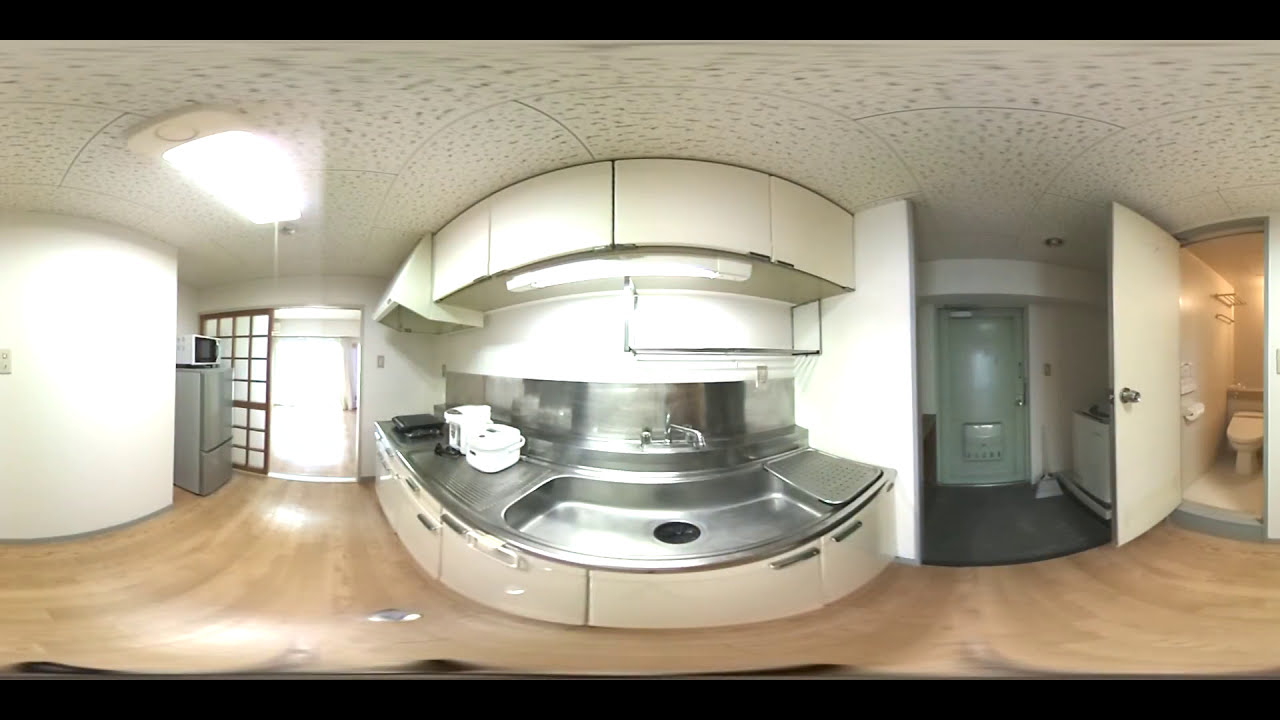This image depicts a wide-angle view of a predominantly white kitchen area that appears to be part of an apartment or house. The kitchen features light brown hardwood floors and a white ceiling scattered with beige spots. Central to the scene is a stainless steel sink with accompanying white small appliances, such as coffee makers or buckets, positioned on the steel counter. Cream-colored pantry cupboards or shelving spaces are situated above the sink, contributing to the overall white theme of the kitchen, including the walls and cabinets.

On the far right side of the kitchen, an open door reveals a bathroom, identifiable by a roll of toilet paper and a white toilet. Between the kitchen and the bathroom is a shut sage-green door, possibly leading to a laundry room, with a white broom propped against the adjacent wall. To the far left, a stainless steel refrigerator stands beside a black and white microwave, in front of a room with Japanese-style sliding doors. The wide-angle view adds a slightly distorted effect, making the central kitchen area appear to bulge slightly. The apartment seems sparsely furnished, suggesting it might be new or up for sale.